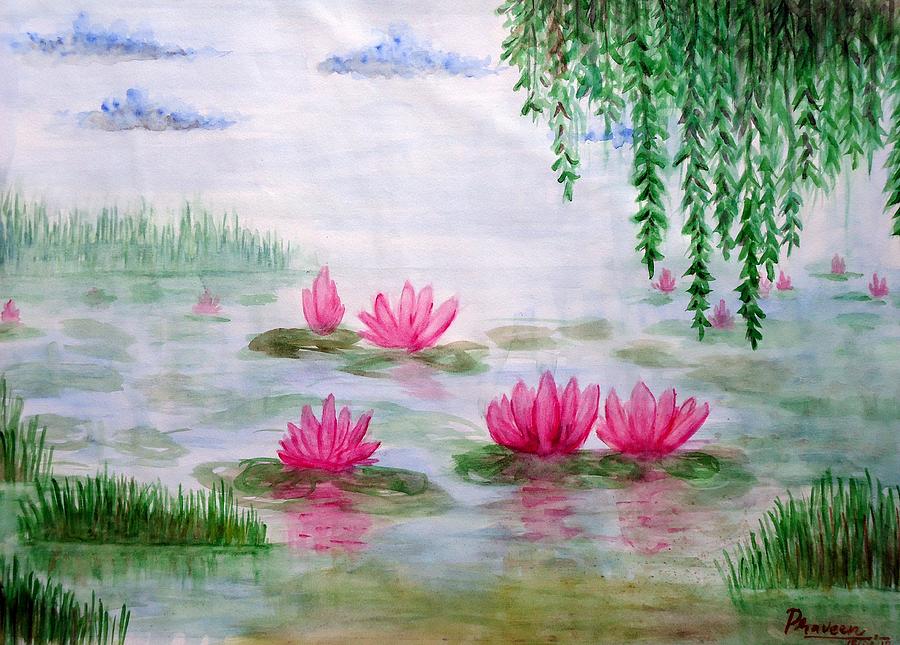This beautifully painted watercolor image features a serene pond brimming with life and color. At the heart of the scene, numerous pink lotus flowers bloom vibrantly atop clusters of lily pads, casting delicate shadows on the surrounding water. Green plants and patches of grass emerge from the pond's surface, while more lush foliage, possibly from a hanging willow tree, drapes gracefully into the frame from the top right corner. The sky above is a subtle grayish-blue, adorned with blue-highlighted clouds, which contrast with the vivid natural elements below. The artist has skillfully captured reflections and shadows, adding depth to the composition. In the bottom right corner, the artist's signature provides a final touch, anchoring the viewer's eye in this tranquil, nature-inspired scene.